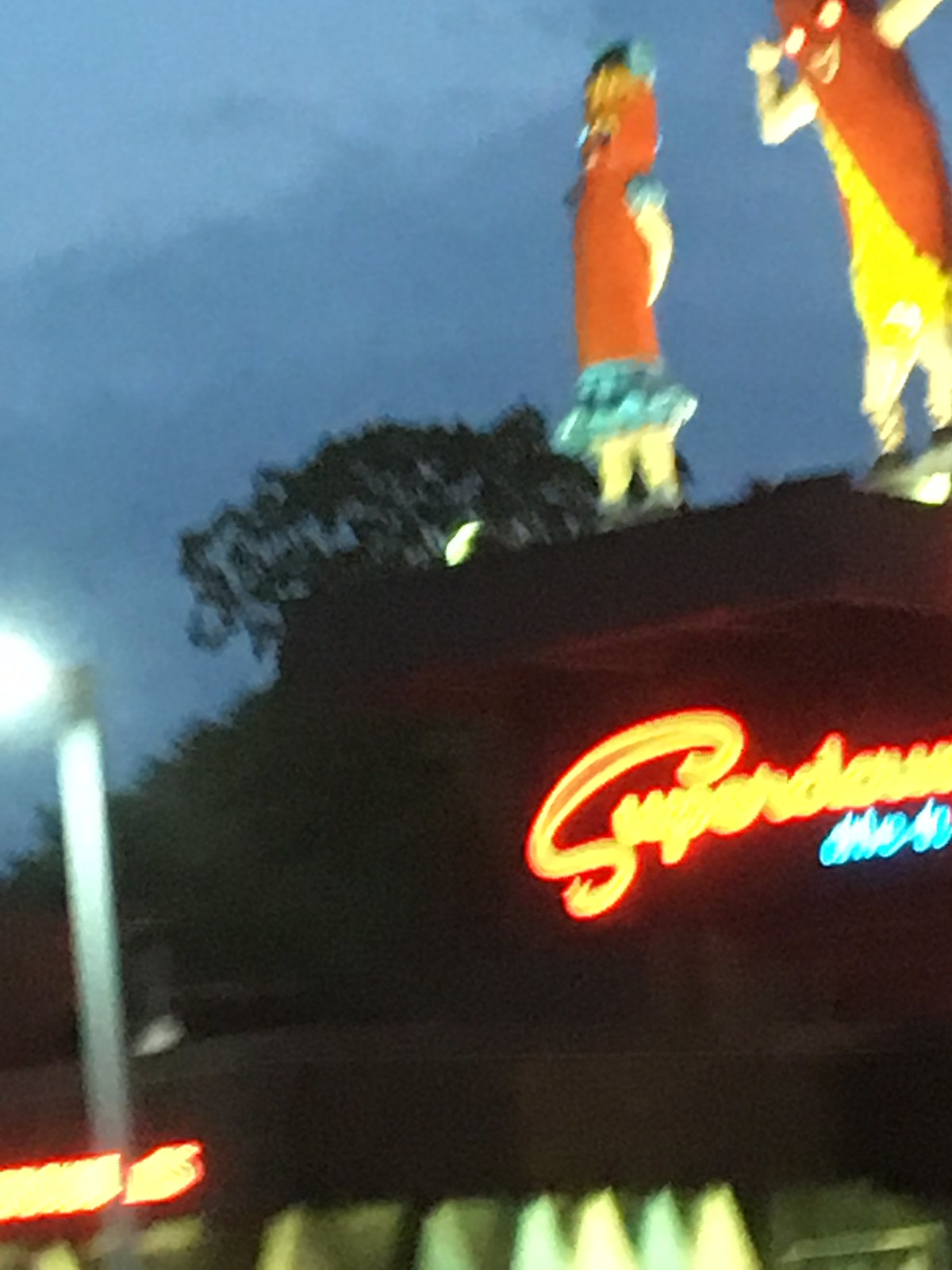The image is a blurry, out-of-focus photograph taken outside a building that appears to be a restaurant, possibly named “Super Down” or something similar. The establishment’s name is partially visible in orange neon cursive lettering, though slightly cropped and difficult to decipher. Below it, some blue and white neon lights are present, spelling out additional text that remains unreadable. The scene is set during the evening, under a dark gray-blue sky. 

On top of the building, two whimsical hot dog figures are displayed. The first figure, resembling a female hot dog, has white legs, is dressed in a blue skirt with matching ruffles on her shoulders, and wears a blue bonnet over curly blonde hair. The second figure, which appears to be a male hot dog, sports a yellow garment that looks like overalls or a one-shoulder leotard, with red eyes, a white grin, and white arms raised near its head. Surrounding the structure, there are clouds in the sky and a leafy tree rising above the building, adding to the evening ambiance.